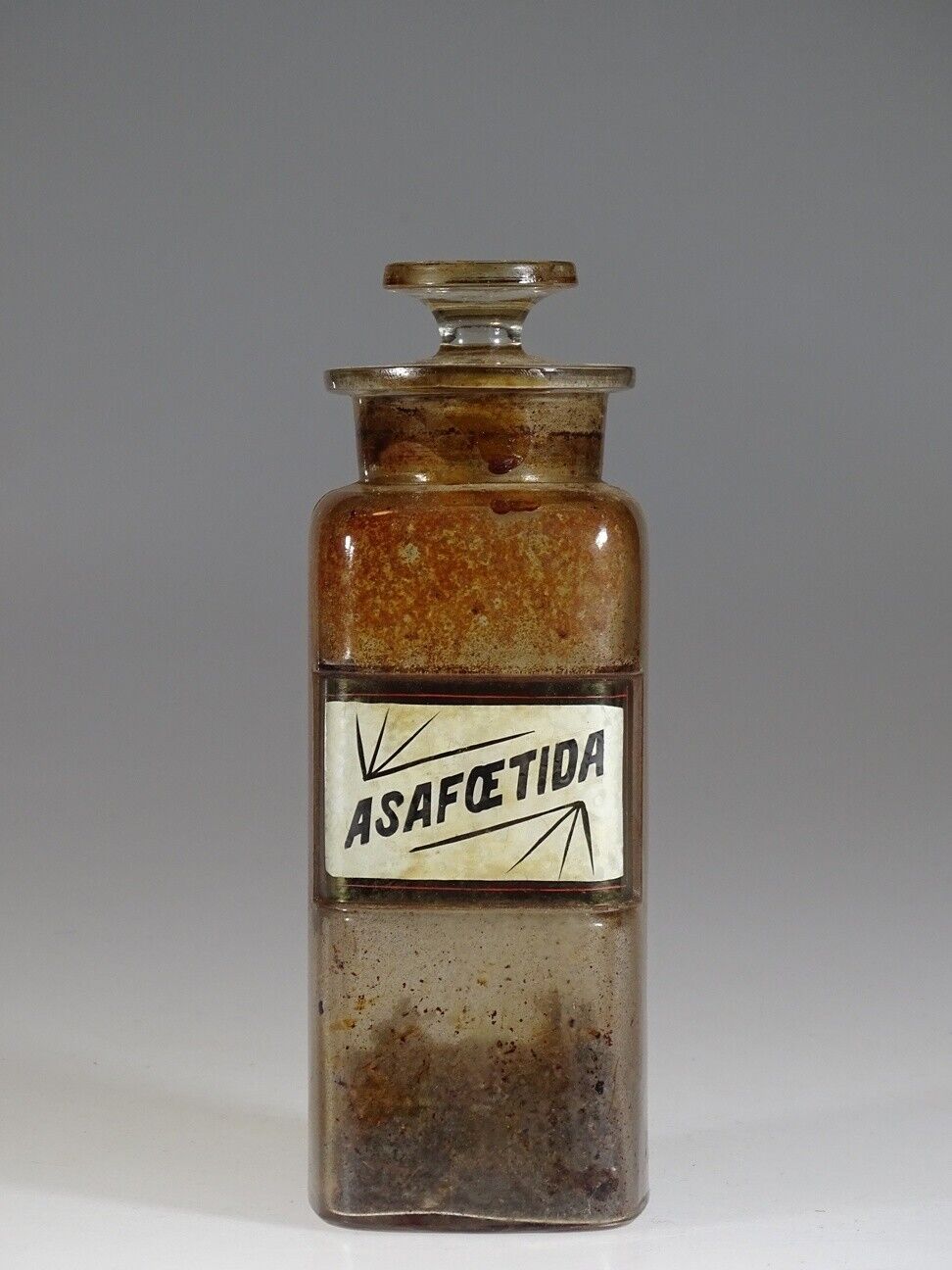The image portrays an antique glass apothecary bottle, likely from the Victorian era, occupying the center and approximately 75% of the photograph. Set against a dark gray background that gradually lightens to a whitish base, the bottle casts a faint shadow to its right. The timeworn glass bottle features a stopper at the top and showcases signs of wear, with a brownish tint starting from the stopper downward, possibly stained by its contents over time. A prominently placed, black-bordered label with decorative lines above and below the wording reads "Asafoetida," featuring an unusual combined "O-E" character in the middle. This label sits diagonally on the bottle's surface. The jar appears dusty and dirty, with visible residue on the interior: a mix of brown gunk near the top and what looks like dirt or old spices settled towards the bottom, suggesting it has not been cleaned recently. The overall appearance conveys a sense of historical usage and neglect.